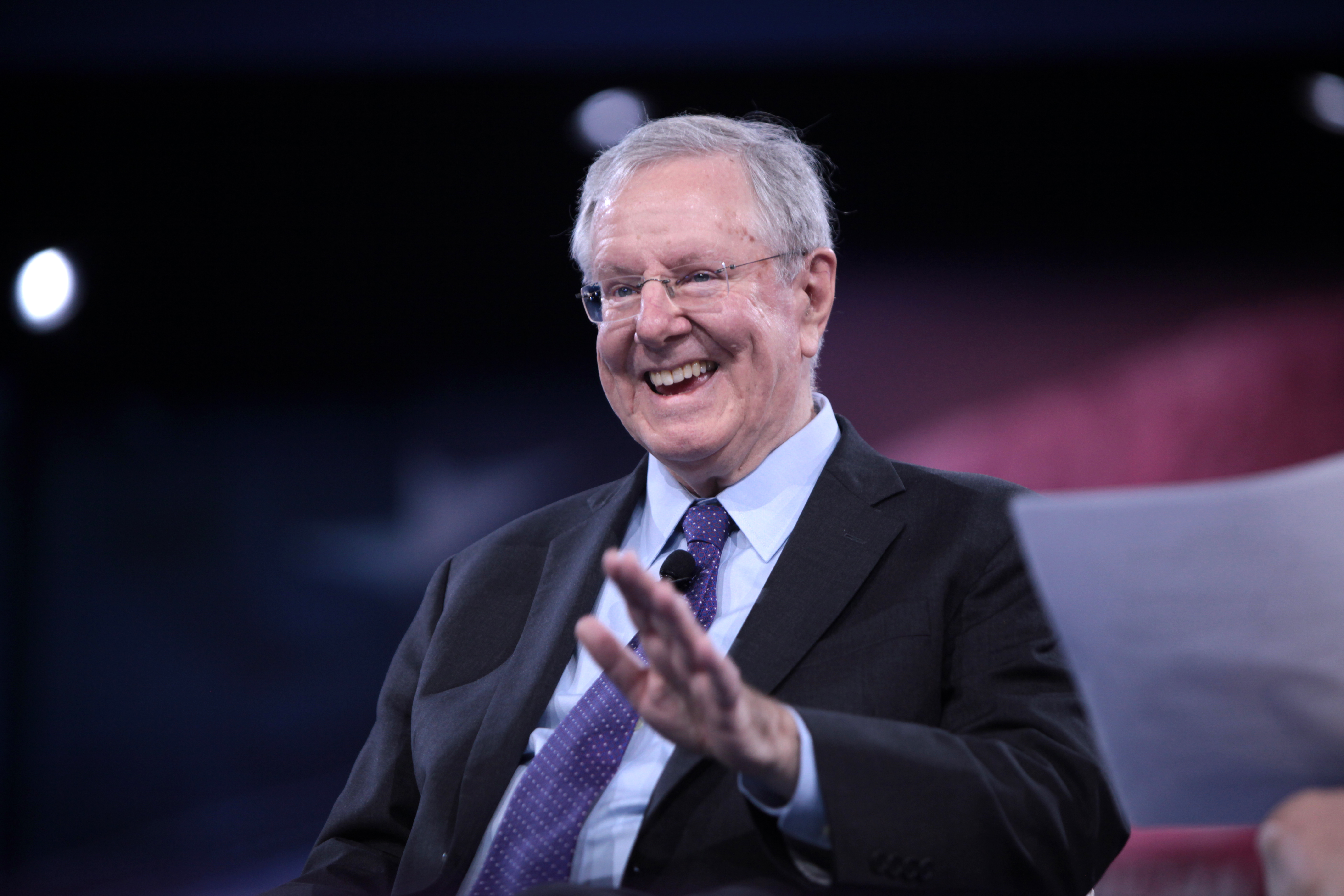The photograph features an older gentleman, likely over 65, with white hair and a fair complexion. He is the main focus of the image, which has a blurry background consisting of a mix of black and faint red with a light white hue near the center and a gray segment resembling a piece of paper on the right. The man, exuding a distinguished and professional appearance, is dressed in a black jacket with large collars, a white collared shirt, and a blue tie adorned with white polka dots. He is also wearing spectacles and a microphone is attached to his tie. The gentleman is captured mid-laugh with his mouth open and his left hand raised, projecting a joyful and engaging presence.